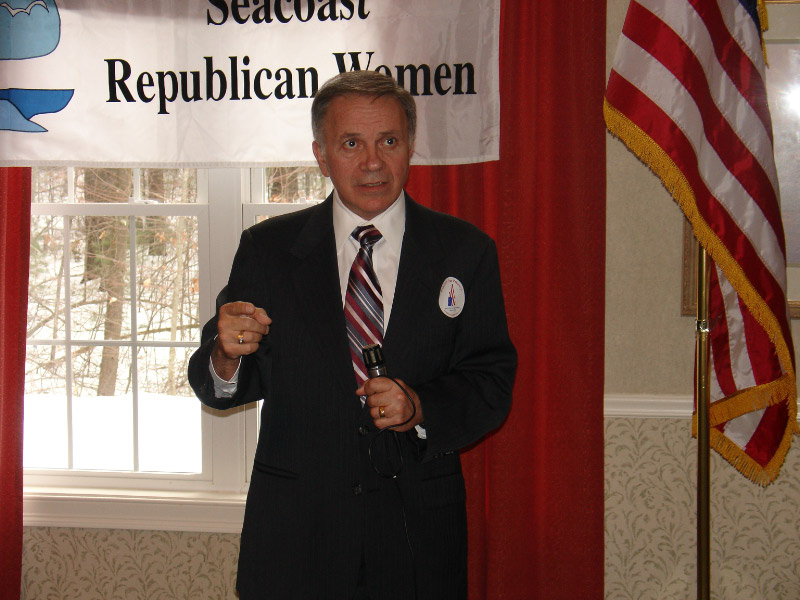In this photograph, an older Caucasian gentleman, likely a politician around 55 to 60 years of age, is captured mid-speech. He stands poised in a dark gray or black suit, complemented by a white button-down shirt and a striking striped tie featuring dark red, blue, and white hues. A notable feature is the white sticker or badge with an insignia on the left side of his chest (our right). The man, who has darker gray hair styled neatly reminiscent of a newscaster's cut, appears serious and is gesturing with his left hand while firmly holding an older-style microphone at waist level with his right hand. His eyes are directed towards the upper right part of the frame as if addressing someone or something slightly above him.

In the background, a large window reveals a snowy, leafless winter scene, enhancing the cold, barren atmosphere outside. Above this window is a prominent banner reading "Seacoast Republican Women," flanked by red curtains. An American flag with gold fringe stands to the right on a golden pole, positioned in front of a wall adorned with a photograph or painting. The overall setting and his serious demeanor suggest that he is addressing a significant issue or responding to a question, likely in a formal gathering.